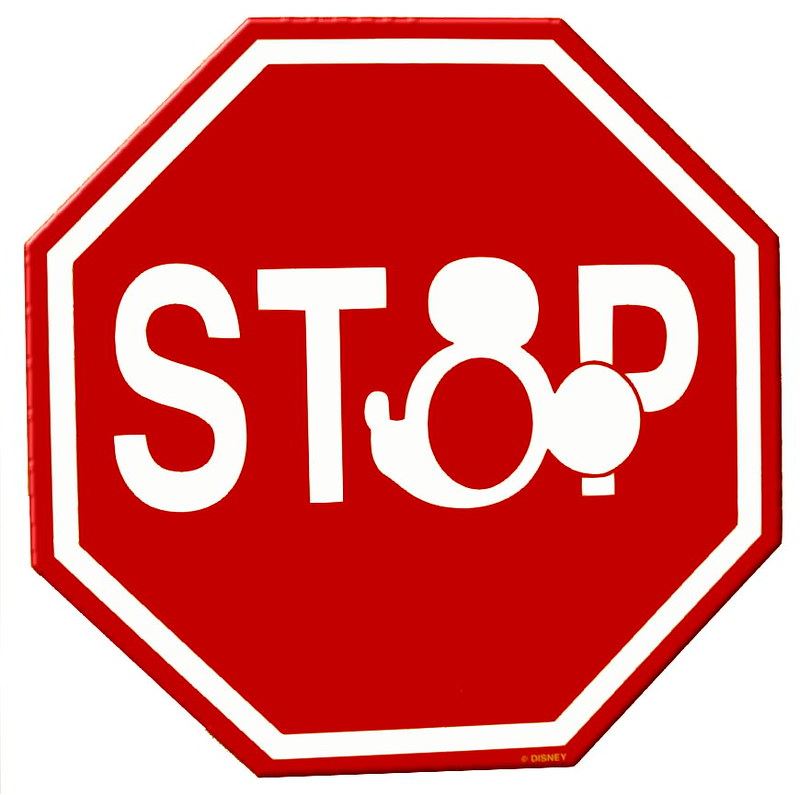The image features a standard octagonal stop sign set against an entirely white background. The stop sign's unique design replaces the letter "O" in "STOP" with a white silhouette of Mickey Mouse's head. This includes his iconic features: the mouse ears (one positioned at the top right and the other overlapping the letter "P"), his snout, and a nose that faces left. The sign has a two-layered border, with a white inner border followed by a red outer border. In the bottom right corner, the word "Disney" is prominently displayed in golden yellow text.